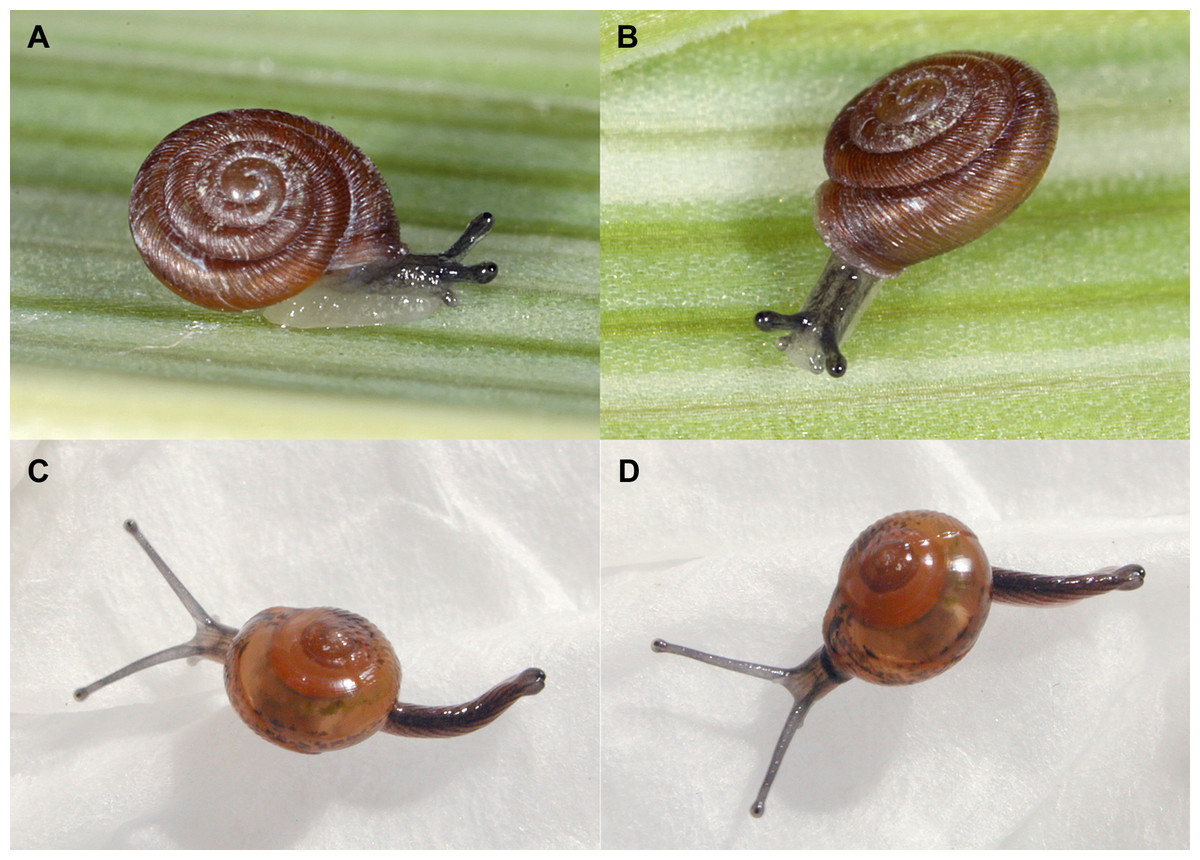The image is a rectangular collage divided into four labeled sections featuring snails, with two images on the top row and two on the bottom row. 

In section A (top left), a large snail with a black body, black antennae, and a brown swirly shell is captured side-on, moving rightward on a light green leaf background, leaving a slime trail. 

Section B (top right) presents the same snail from an overhead view, heading towards the lower left corner, also on a green leafy backdrop.

Section C (bottom left) features a smaller snail with a translucent head, antennae, and an orange shell, moving directly west on a white background. This snail displays a worm-like tail trailing behind it.

Section D (bottom right) shows a similar smaller snail to section C, moving towards the lower left, depicted with a white background from an overhead diagonal angle.